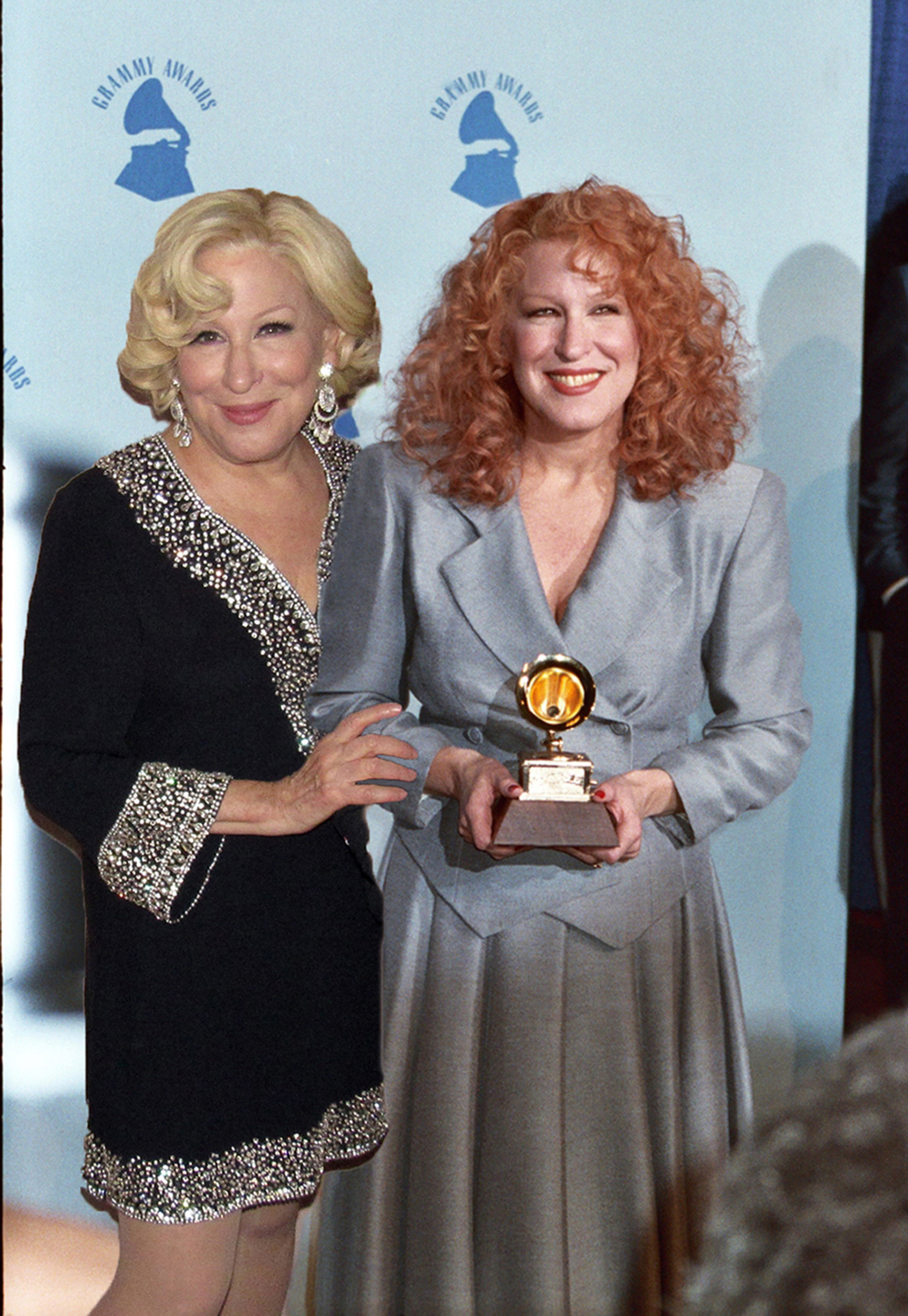This photograph features two women side by side, both appearing as Bette Midler, though in different attire and seeming to be at different stages of her career. The Bette Midler on the left, a white female with short blonde hair, is adorned with long, diamond-studded earrings. She is wearing a long black dress intricately decorated with diamonds and silver detailing around the collar, sleeves, and hem. Her expression shows a warm smile, though you cannot see her teeth.

Standing next to her is another depiction of Bette Midler with curly red hair and bright red lipstick. This younger version is dressed in a sophisticated ensemble comprising a gray suit jacket paired with a long, matching skirt. She is holding a Grammy award and smiling broadly, showing her teeth. The setting features a blue backdrop with a blue Grammy logo and the text "Grammy Awards" prominently displayed above.

The image gives the appearance of a photoshopped creation where the older Bette Midler is seemingly congratulating the younger Bette Midler on her Grammy achievement, blending nostalgia with celebration.